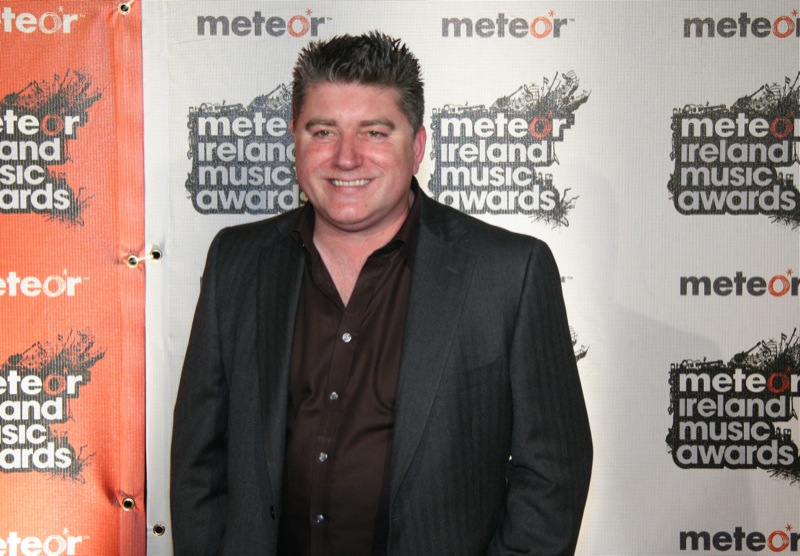The photograph captures a slightly overweight, white male standing in front of a backdrop adorned with the "Meteor Ireland Music Awards" logos. The man is visible from the waist up, smiling with a slight tilt to the right, his short, spiked hair accentuating his clean-shaven face. He is dressed in a maroon button-up shirt, with the top button left open, revealing a bit of his neck. Over this shirt, he wears a dark grey, striped suit jacket, left unbuttoned. His hands rest naturally at his sides, with elbows slightly bent. The backdrop behind him features repeating logos of "METEOR" in bold black text, with a distinctive red "O," and below it, the phrase "Meteor Ireland Music Awards" in white text with a black border. The backdrop's colors alternate between white and orange panels, held together with white zip ties, which are visible in the image. His shadow is cast upon the backdrop, adding depth to the scene.